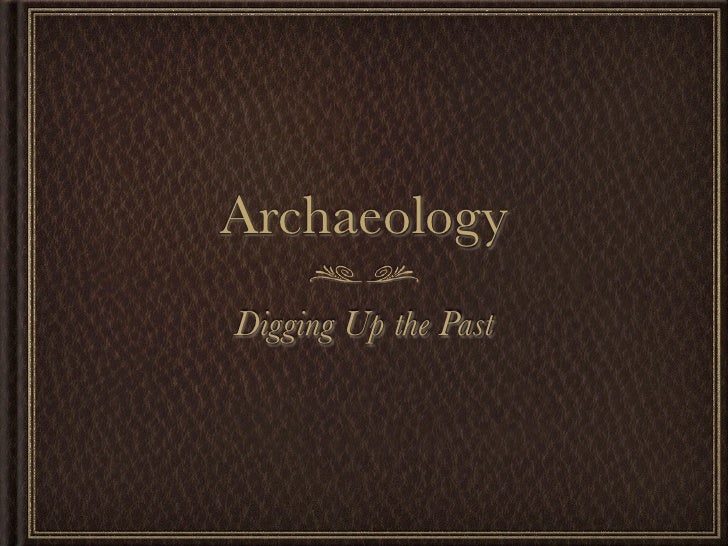The object in question is the cover of a book, characterized by a brown, leather-bound appearance that features a distinctive textured pattern resembling scales. Surrounding the perimeter of the cover is a dual-framed golden border: an outer thick gold rectangle and an inner thinner gold rectangle. At the center, the title "Archaeology" appears in standard print, rendered in gold lettering, with the subtitle "Digging Up the Past" beneath it in italicized script. Additionally, the space between the title and the subtitle is adorned with decorative flourishes that resemble floral patterns or heads of wheat. The book cover as a whole is wider than it is tall.